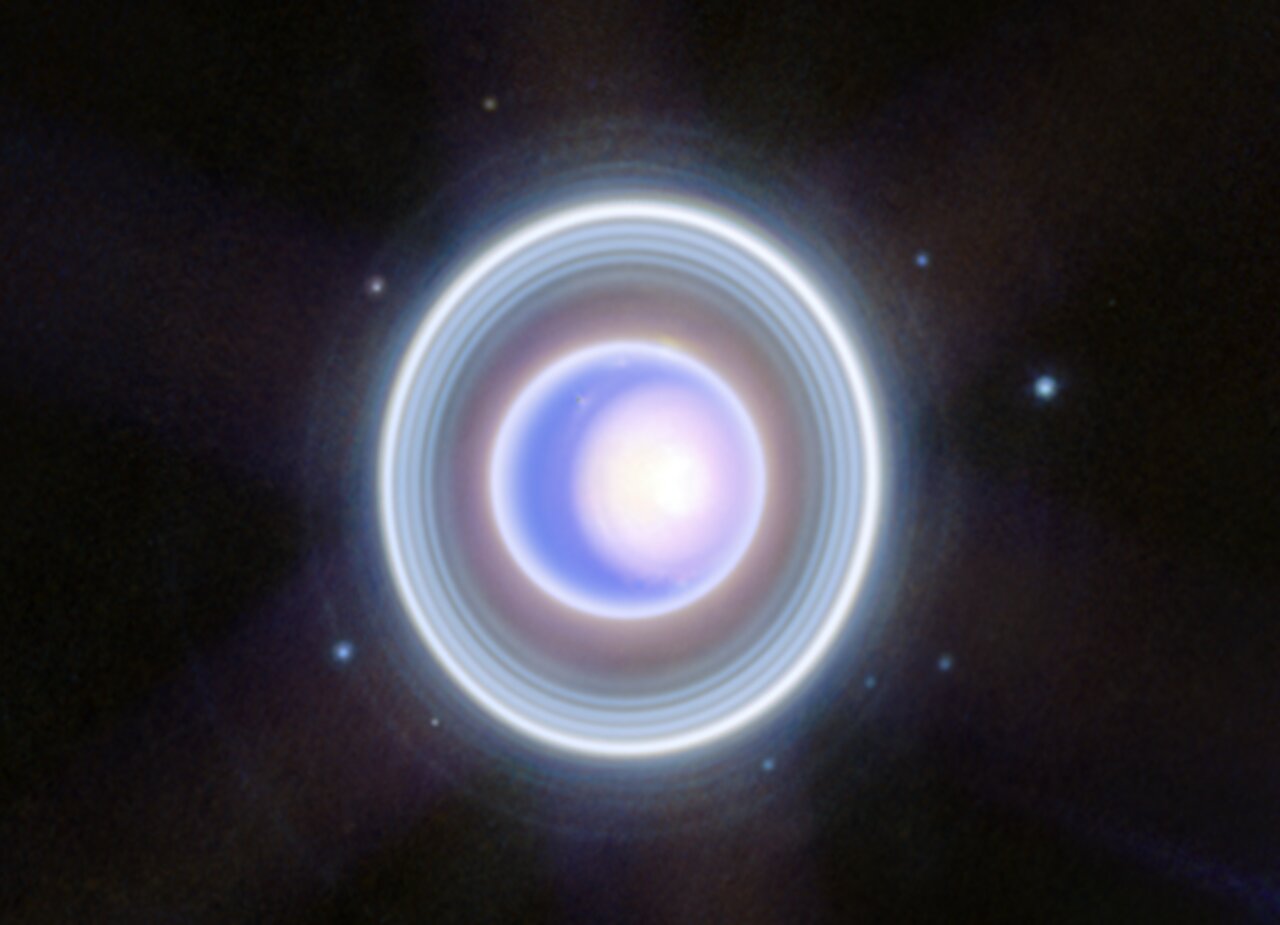In the middle of a black, star-dotted cosmos stands a striking azure planet enveloped by five distinct rings. The planet is illuminated with a faint white glow, enhanced by a light purple hue towards its center. The following rings exhibit varying shades of blue, with the innermost one exhibiting a white circle that diffuses into a soft purplish tone. Next comes a ring resembling the serene color of the sky but slightly darker. Outside this sphere, the rings transition from purplish black to gray, then to light blue, before culminating in a luminous white ring, and finally a delicate blue hue. The outermost ring, the fifth one, radiates the brightest, appearing almost white. Subtle beams of bluish-purple light extend outwards, interspersed with a sprinkling of white dots, creating a majestic spectacle against the dark expanse of space. The arrangement, occupying about half the width of the frame, evokes an ethereal and cosmic grandeur, blending serene colors with the enigmatic allure of the universe.